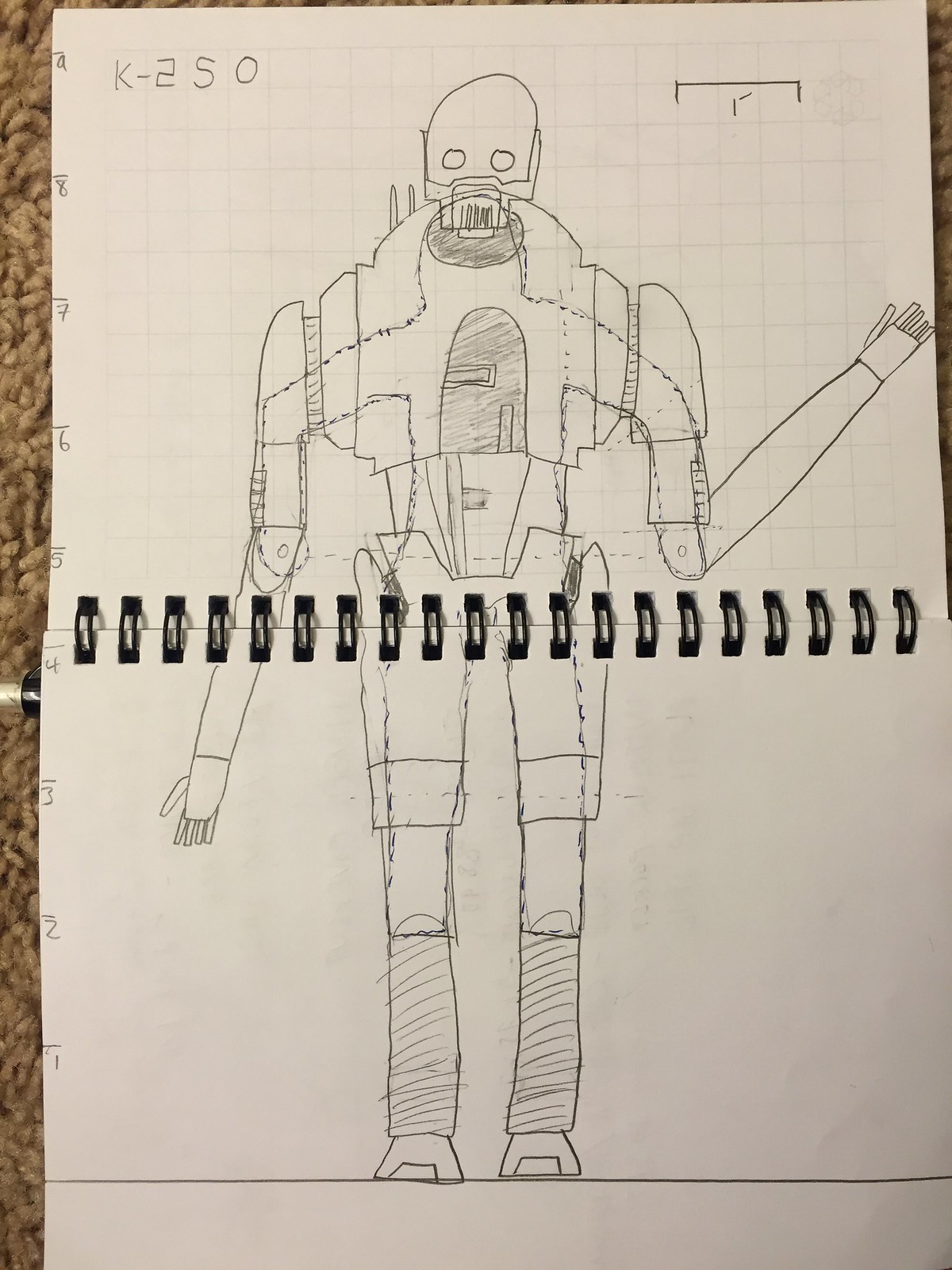This vertical rectangular image depicts a pencil drawing of a robot on graph paper, situated in a notebook held together by double sets of black coils, possibly comb or ring binding. The grid paper, adorned with numbers 1 to 9 on the left margin, occupies the top half of the page, transitioning into blank white paper on the bottom. The robot, labeled "K-250" at the top left corner, stands along a line at the base of the graph section. The character features squarish thighs, hips, legs, and feet, along with boxy arms — one bent upward displaying fingers. Its upper body is distinguished by a round head with indistinct eyes, a flat jawline, a semicircular chest tapering into a detailed, segment-riveted torso. Accompanying elements include a small scale indicator demonstrating three grid squares as one foot, and a light brown, oatmeal-like carpet visible around the paper's edges, further highlighting the intricate yet classic design of the robotic figure.